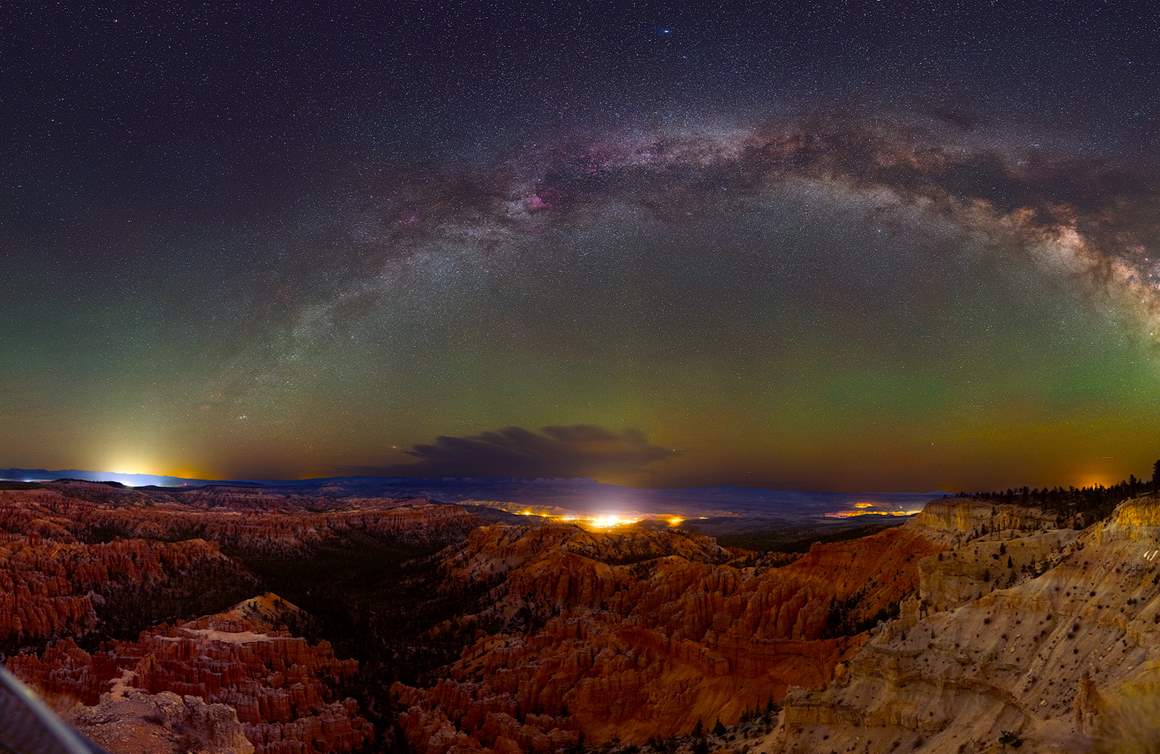This stunning night-time photograph captures a mesmerizing view of a starry sky, dominated by the Milky Way arcing gracefully overhead. The top two-thirds of the image are a tapestry of stars against a dark purple to deep blue sky. The Milky Way appears as a curved band of light, resembling a celestial rainbow of glowing, gaseous clouds. The photo is set just after dusk, with a gentle gradient of green and gold light lingering on the horizon, indicating residual sunlight. 

Below this vivid celestial display lies a rugged, red-orange rocky landscape reminiscent of Bryce Canyon or Utah's iconic canyons. The rocky mountains and cliffs are bathed in rust and dark orange hues, adding depth and texture to the scene. Scattered across the lower part of the image and near the horizon are pockets of light, likely emanating from distant human settlements, giving the impression of tiny glowing towns. Additionally, some trees can be seen in the right background, subtly illuminated by the ambient light.

The overall composition of the photograph, taken from an elevated vantage point, showcases the harmonious contrast between the natural wonders of Earth and the mysterious beauty of the universe.